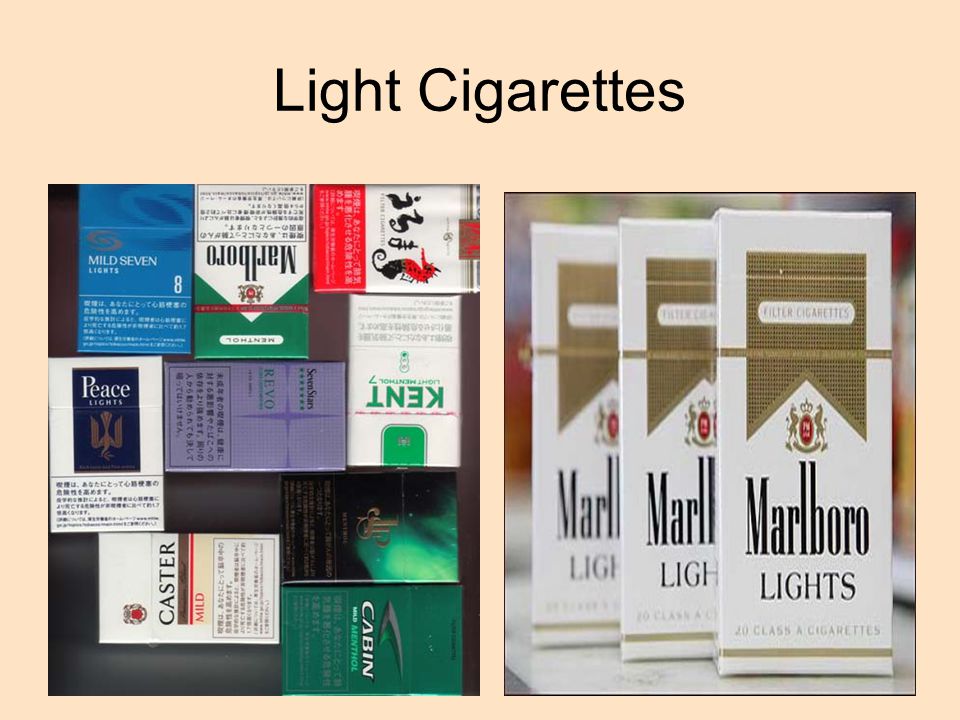The image is set against a light peach or cream-colored background and resembles an advertisement or PowerPoint slide. At the very top, the text "Light Cigarettes" is prominently displayed in black font, with the first letter of each word capitalized. The image is divided into two sections: the left side showcases a variety of cigarette packs, and the right side features three packs of Marlboro Lights.

On the left side, there are nine different cigarette packs arranged haphazardly, with some upright, some upside down, and some sideways. The packs are in various colors such as green, white, red, blue, and lilac, reflecting different brands. Notable brands include a blue pack of Mild 7 Lights with white text, an upside-down Marlboro with a green top and white bottom, a white and red pack with a seahorse logo, an upside-down Kent with green text, a lilac-colored pack labeled Revo, and a white pack with a blue rectangle reading Peace. Other visible brands include Caster and Cabin, with the latter packaged in mostly green.

The right side of the image presents three identical Marlboro Lights packs positioned vertically in a staggered row. These packs are primarily white with gold at the top. The branding features "Marlboro Lights" in black text and "20 Class A Cigarettes" in gold below it, along with a distinct gold stripe towards the bottom of the box.